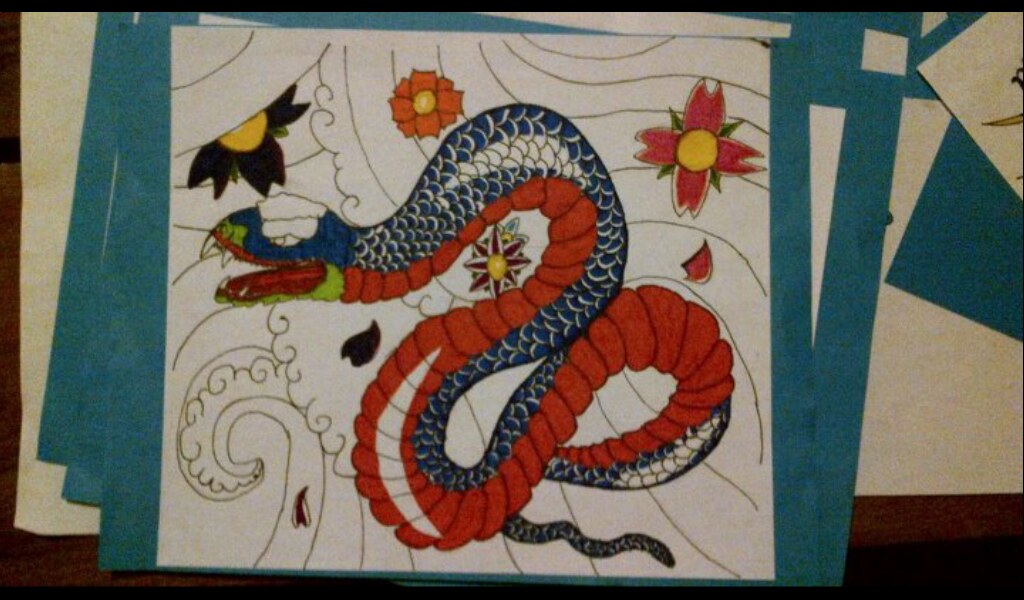The photograph showcases a collection of hand-drawn artworks, meticulously layered on top of one another on a table. The central piece features a detailed illustration of a serpentine creature, potentially a snake, adorned with dragon-like scales running along its back. This focal artwork is mounted on blue construction paper, with hints of other similar pieces peeking out from underneath, indicating a series of these intricate drawings.

The snake itself is a vibrant amalgamation of colors and patterns. The head of the snake is predominantly blue, transitioning to green towards the lower jaw. The body is embellished with blue and white scales, while the underbelly sports accents of orange and red, resembling both scales and worm-like textures.

Surrounding the snake is a whimsical array of elements, including what appear to be fringe or lace-like curls in an array of colors, adding a decorative flair reminiscent of ornate curtains. The background is further enriched with various floral motifs: a prominent black flower featuring a red dial at its center, alongside other flowers in hues of orange and red.

Overall, the artwork exudes a lively and imaginative spirit, blending detailed natural elements with fantastical design, resulting in a visually captivating piece.